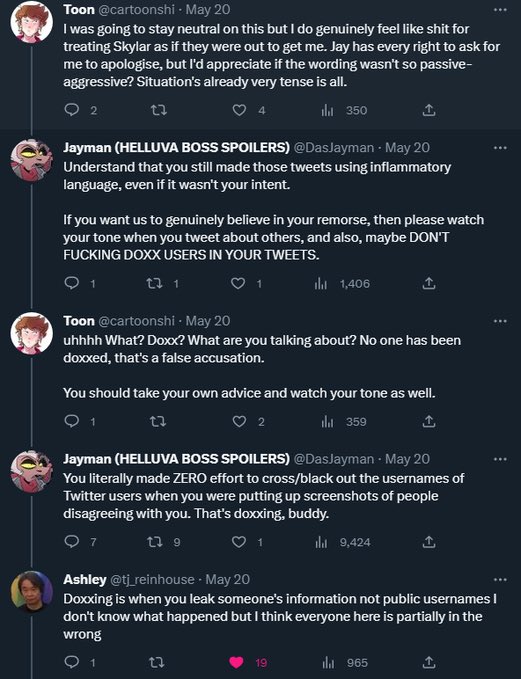On a dark gray background, the image showcases a chat interface featuring a dialogue exchange. The chat page belongs to "Jay Man" and includes a user profile picture of a cartoon character. The primary message from the user reads: "I was going to stay neutral on this, but I genuinely feel bad for treating Skylar as if they were out to get me. Jay has every right to ask for an apology, but I would appreciate if the wording wasn't so passive-aggressive. The situation is already very tense."

Below this, another message from "Jay Man (H-E-L-L-U-V-A All Spoilers)" highlights: "Understand that you still made those tweets using inflammatory language, even if it wasn't your intent. If you want us to genuinely believe in your remorse, then please watch your tone when you tweet about others. And also, DON'T F-U-C-K-I-N-G DOX other users in your tweets."

The interface includes several icons: a chat bubble with the number two, a heart with the number four, and a bar graph displaying the number 350.